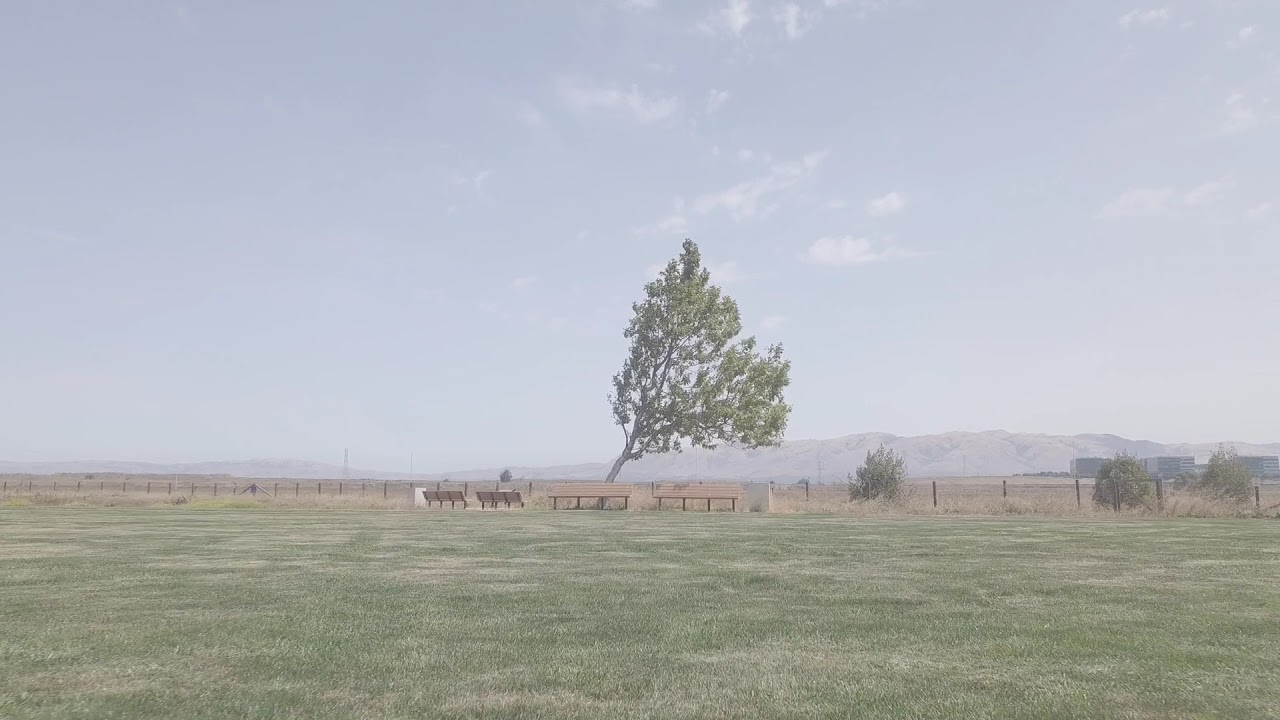The image depicts a sprawling, open grassy field mottled with patches of green and yellow, suggestive of seasonal change. Dominating the central foreground is a large tree with a thick trunk, heavy with green needles, that leans distinctly towards the right, partially revealing the hazy blue sky and thinly scattered clouds behind it. Arranged in front of this tree are two sets of benches painted an orange metal color, accompanied by two additional bench-like structures with wooden backrests that almost blend into the natural surroundings. Off to the side, the field transitions into a fence line formed by wooden posts that runs horizontally across the image, flanked by three smaller, verdant trees. In the background, to the right, the landscape extends into a grayish-brown mountain range under a lightly dust-filled sky, with distant hints of brown hills, electrical towers, and barely discernible high-rise buildings, suggesting the outskirts of an office park.